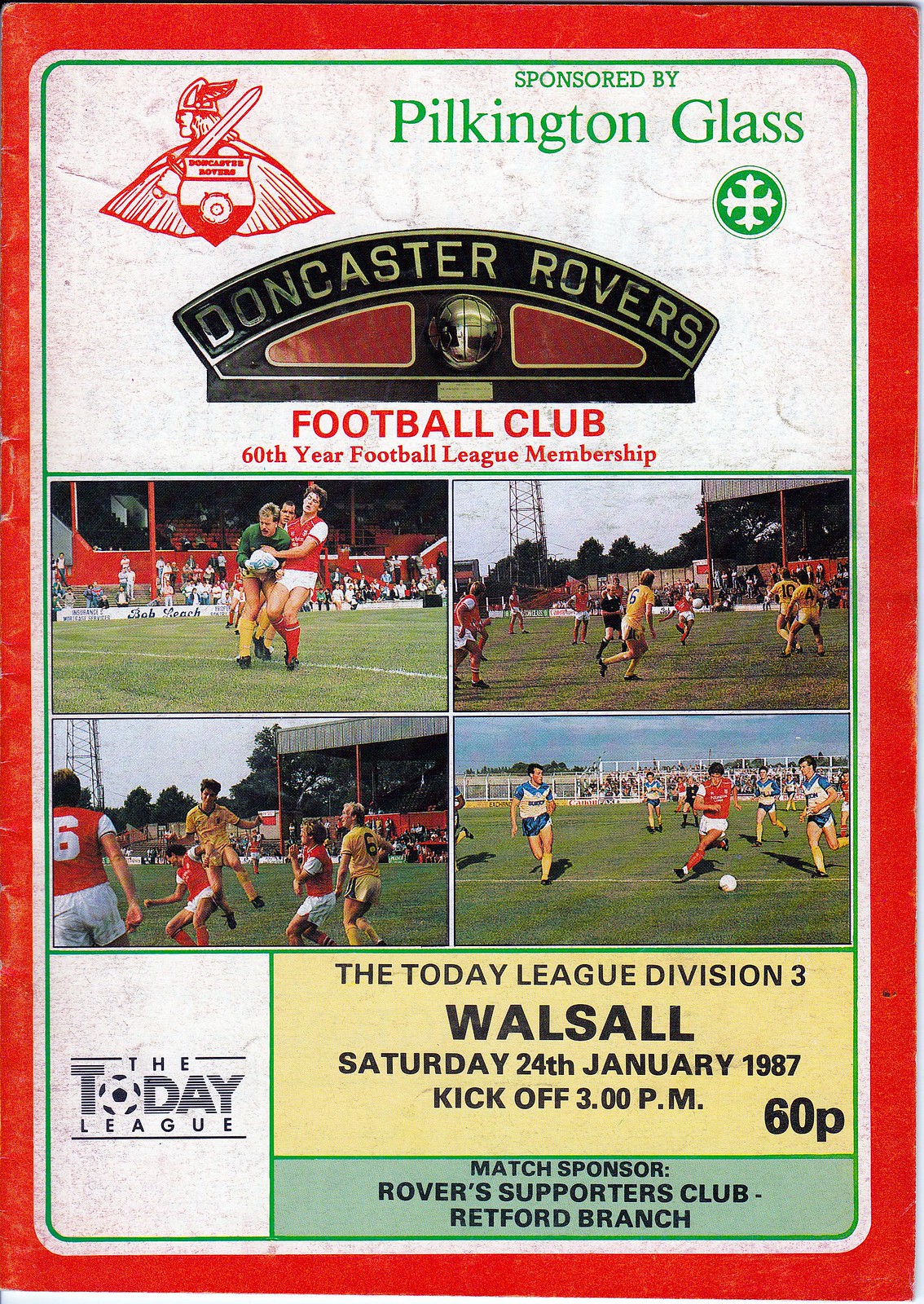The image is the cover of a soccer magazine or program for a sports game, prominently featuring multiple snapshots of soccer action in a collage format, showcasing the Doncaster Rovers Football Club. The cover commemorates the club's 60th year in the Football League. The collage consists of four photos depicting various game moments, consistently featuring the Doncaster Rovers playing against different teams. The primary text at the top reads "Pilkington Glass Doncaster Rovers Football Club 60th Year Football League Membership," highlighted in gold lettering on a black background. The left side includes an image of a Viking holding a sword over his shoulder, and a crest or shield which partially reads "Casters." Below the collage, it says "The Today League Division III Walsall, Saturday, 24 January 1987," with a kickoff time of 3 p.m. The event is sponsored by "Rovers Supporters Club, Redford Branch," with an entry price of 60p. Additionally, there is a round emblem containing a gothic cross and the text "Sponsored by Pilkington Glass" appears in green in the upper right corner.